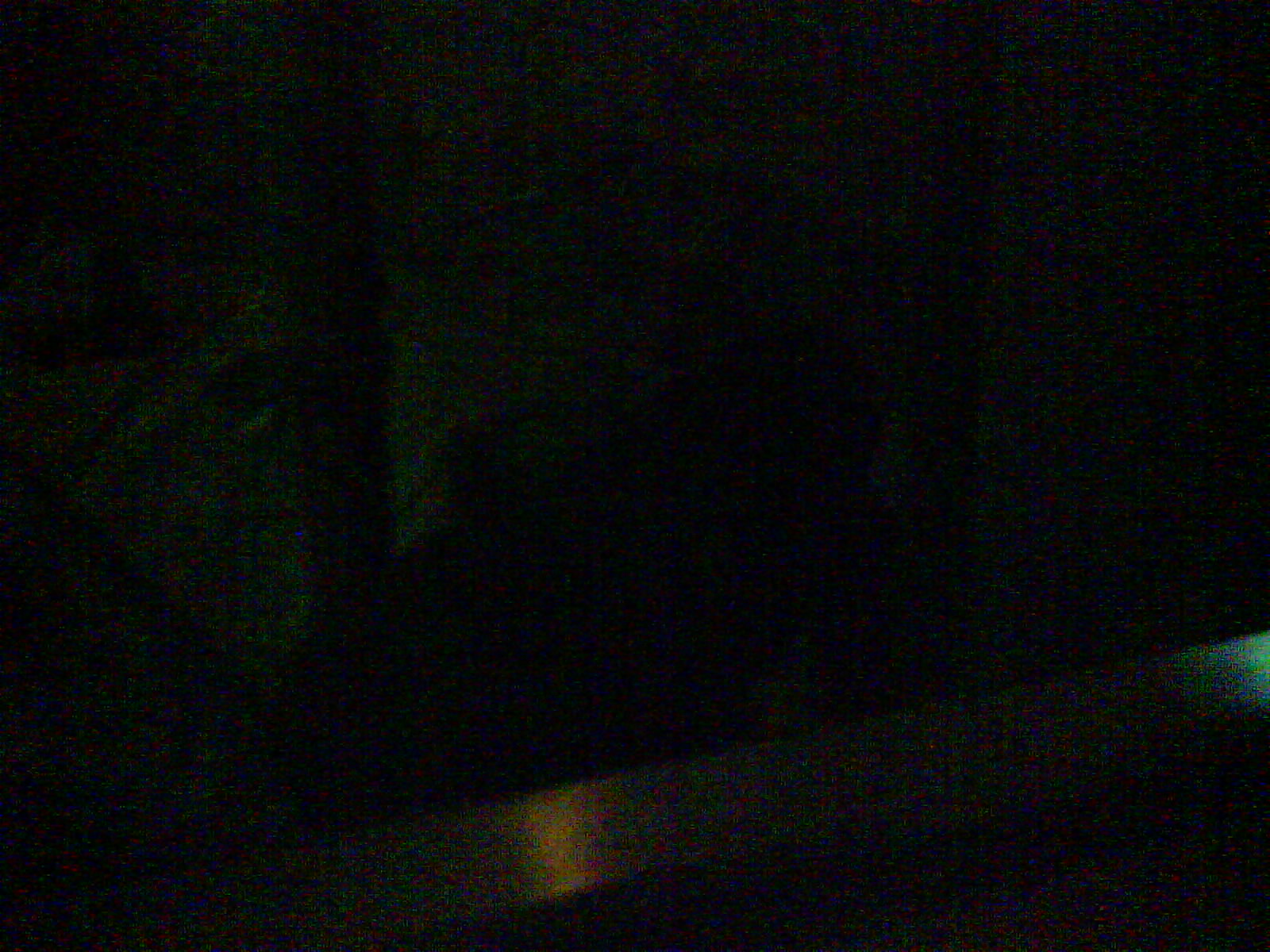This is a photograph captured in extremely low light conditions, resulting in a predominantly black image with a very grainy texture. A faint, diagonal band of lighter color stretches from the lower-left corner upward to about a third of the way up the right side. Within this band, two reflective patches are slightly more visible: an orangey-tan patch roughly halfway across the image and a light blue patch along the right edge. The upper portion of the photograph contains a few indistinct lighter shapes resembling vertical rectangles extending downward from the top. The lack of adequate lighting makes it difficult to discern any specific subject, leaving the content of the photograph ambiguous and heavily obscured by darkness.